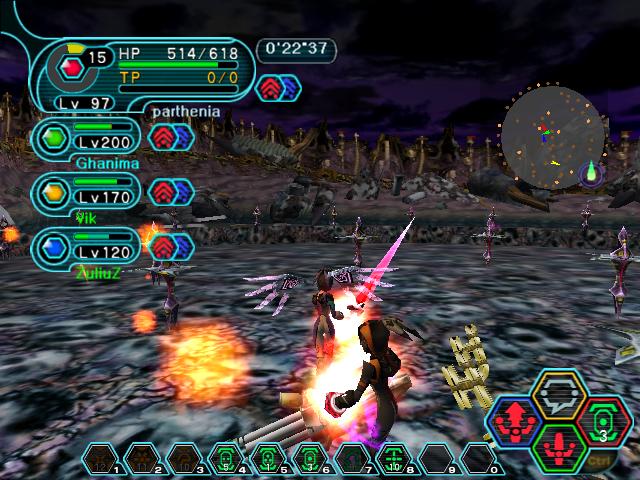This is a vibrant and detailed screenshot from a video game that mixes RPG elements with an eerie visual atmosphere, possibly suggesting a title inspired by classic RPG aesthetics like Final Fantasy. Dominating the bottom of the image is an action bar comprised of ten hexagonal slots, mapped to keyboard numbers 1 through 0. Slots 1, 2, 3, 7, 9, and 0 appear inactive with faded icons, whereas 4, 5, 6, and 8 display active green icons. To the right, four unevenly stacked hexagons feature red and white icons, outlined in various colors including yellow, blue, green, and red.

Set against a disturbing backdrop of gray and white faces with black eye sockets on both the ground and a surrounding wall, the scene provokes a sense of unease. In the midst of this environment are several spinning tops in shades of pink and purple, accented with touches of gold. On the left side of the image is the RPG-style user interface showing the party's information: three members at varying levels—200, 170, and a notably high 1200—all color-coded in blue, yellow, green, and red with green HP bars. The player's health bar, highlighted at the top left, shows 514/618 HP and a TP reading of 0/0, next to a timestamp of '0:22:37'. The listed names, possibly party members or scores, are PARTHENIA, GHANIMA, and AULIU.

The center of the image features two characters amidst combat: one appears to be casting a fireball, and another, more distant figure brandishes a red sword. Above them, there's a large mystical crystal ball with a green teardrop encircled by a purple aura. The scene is bathed in a complex mix of colors, predominantly purple and black, adding to the ethereal, otherworldly feeling of the game environment. In the top-right corner, a mini-map provides navigational context. The overall imagery and layout suggest an intricate, possibly MMORPG setting blending futuristic, fantastical, and unsettling elements.